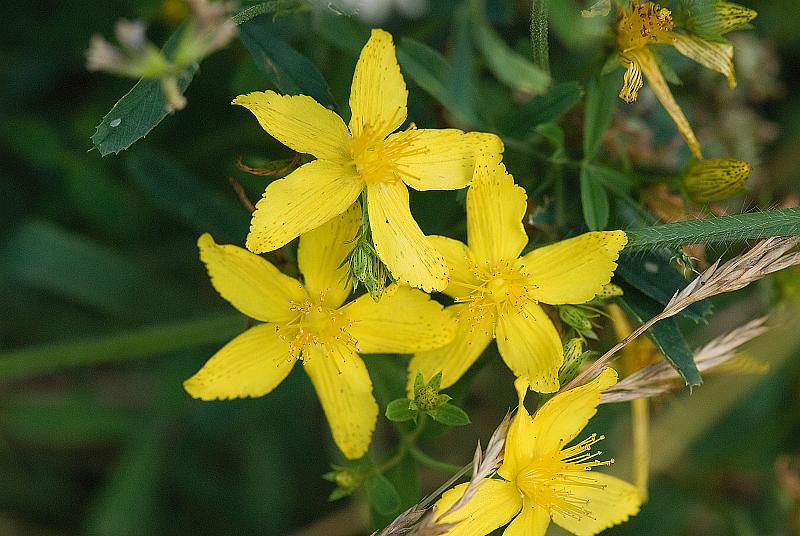The image is a close-up shot of several yellow flowers with detailed focus on their structure and vibrant colors. At the center, three yellow flowers with five petals each form a triangle pattern. Below this grouping lies another yellow blossom, upon which rests what appears to be a piece of wheat. Each flower exhibits prominent reproductive parts, adding to the intricate beauty. In the top right corner, an unopened bud of the same yellow flower hints at future blooms. Surrounding these flowers are a variety of forest green leaves which fade into a blurry background, emphasizing the flowers in the foreground. The overall scene creates a vivid and detailed portrait of these striking flowers, likely similar to dahlias or lilies.